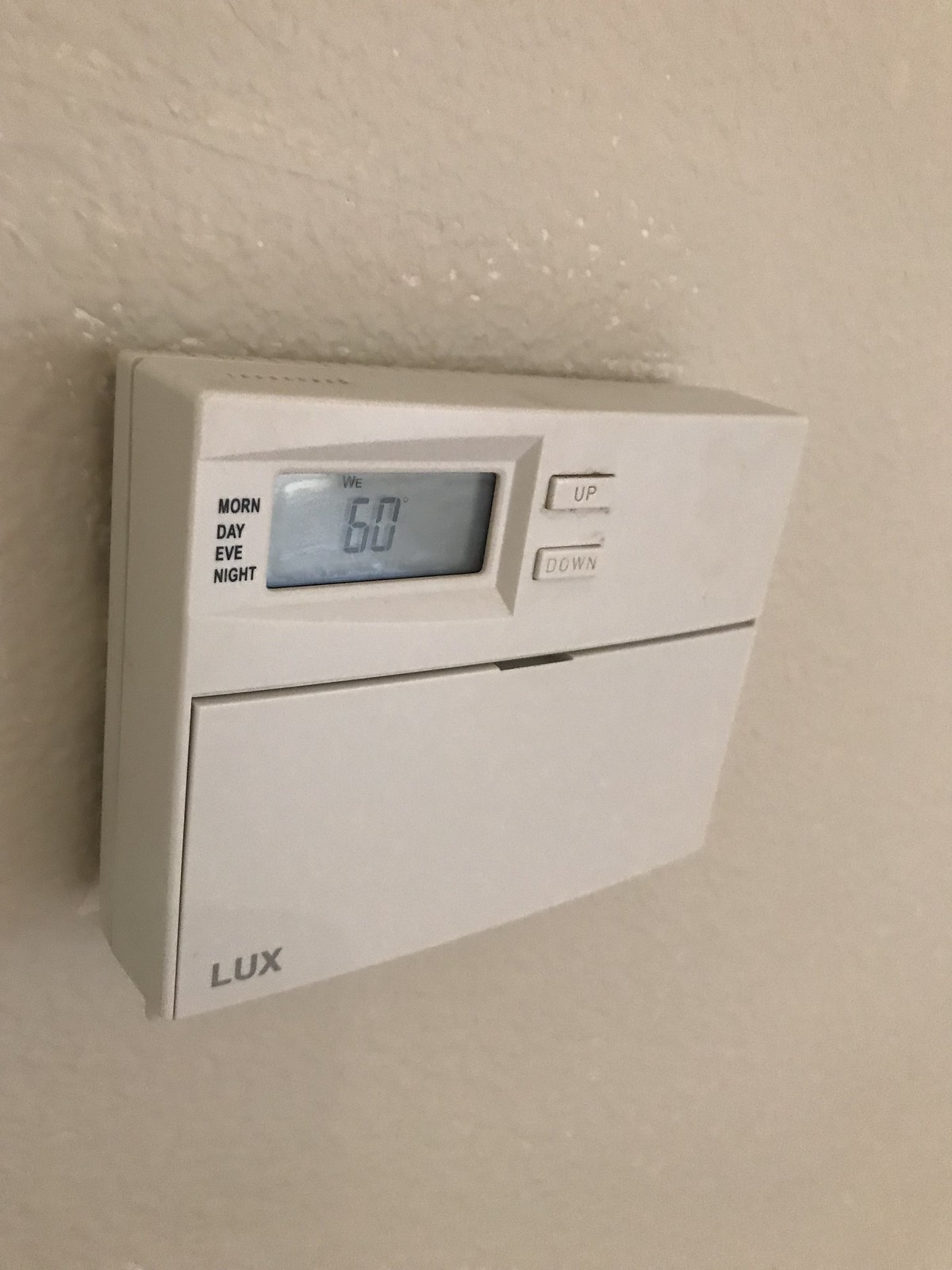The image showcases a digital thermostat mounted on a white wall. The thermostat, which is predominantly white, bears the brand name "Lux" in the bottom left corner, indicating its manufacturer. The device includes labeled sections for different times of the day: "morning," "day," "evening," and "night." The display currently shows a temperature setting of 60 degrees. The thermostat features up and down buttons for adjusting the temperature, with few visible controls on the main interface. A panel appears to be present on the thermostat, likely concealing additional buttons for setting various modes, such as heating or cooling programs for different times of the day. The thermostat's screen, aside from showing the temperature, offers minimal information. The overall design is square and of a moderate size, easily recognizable as a digital thermostat.